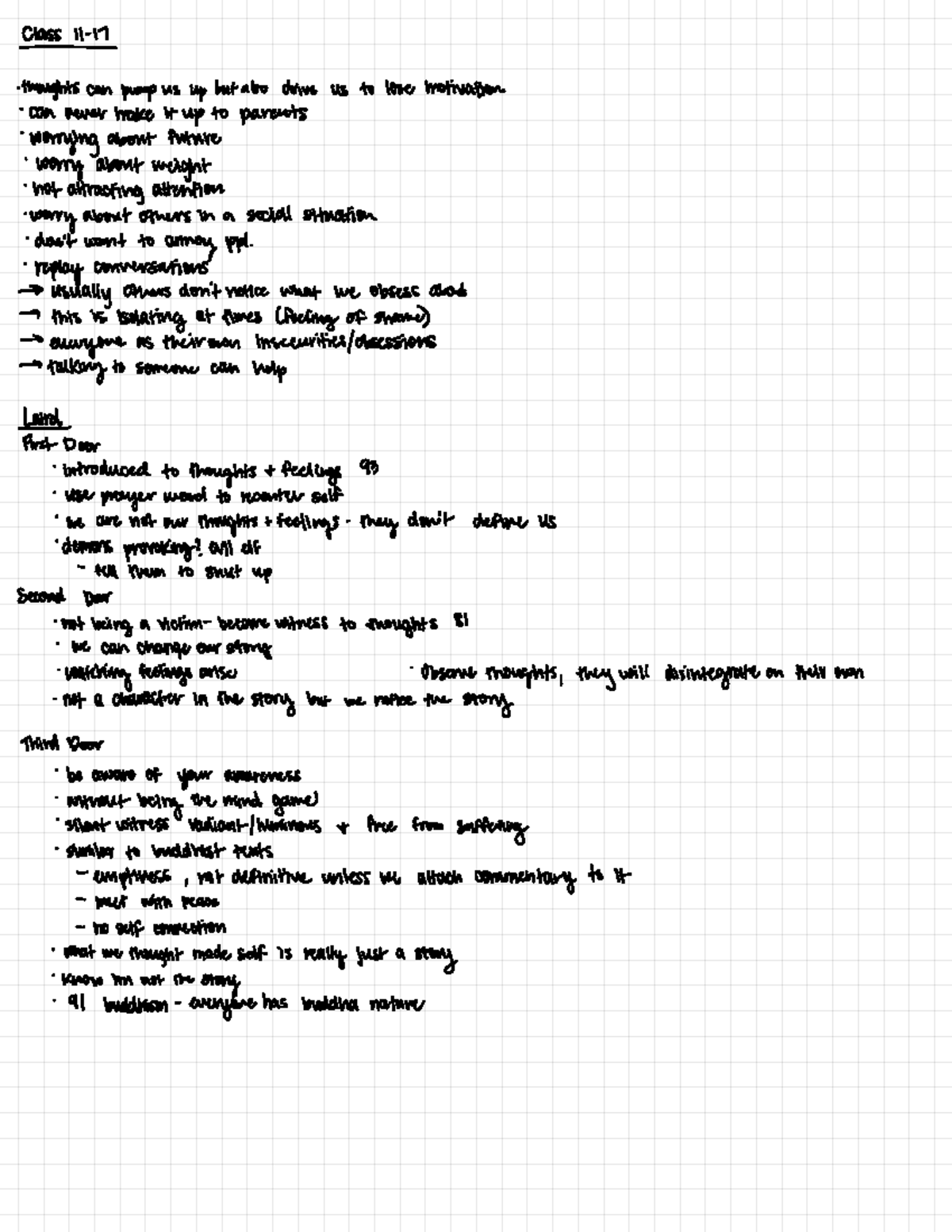This image features a handwritten list separated into two main topics. At the top, it reads "Class 11 - 17." The first section is a series of reflective notes:

1. "Thoughts can pump us up, but also drive us to lose motivation."
2. "Can never make it up for parents."
3. "Worrying about the future."
4. "Worry about weight; not attracting attention."
5. "Worry about others in social situations."
6. "Don’t want to annoy people, reply to conversations."
7. "Usually, what owners don’t take matters, what we obsess about is bothering or boring at times, creating feelings of shame."
8. "Everyone has their own insecurities."
9. "Talking to someone can help."

The second section is titled "Me" and contains a more personal reflection:

1. "First door: Introduced to thought of feeling nine feelings."
2. "93: Use prayer/word to ground or calm herself."

Overall, the list appears to be a deeply personal and contemplative reflection on thoughts, worries, and personal coping mechanisms.